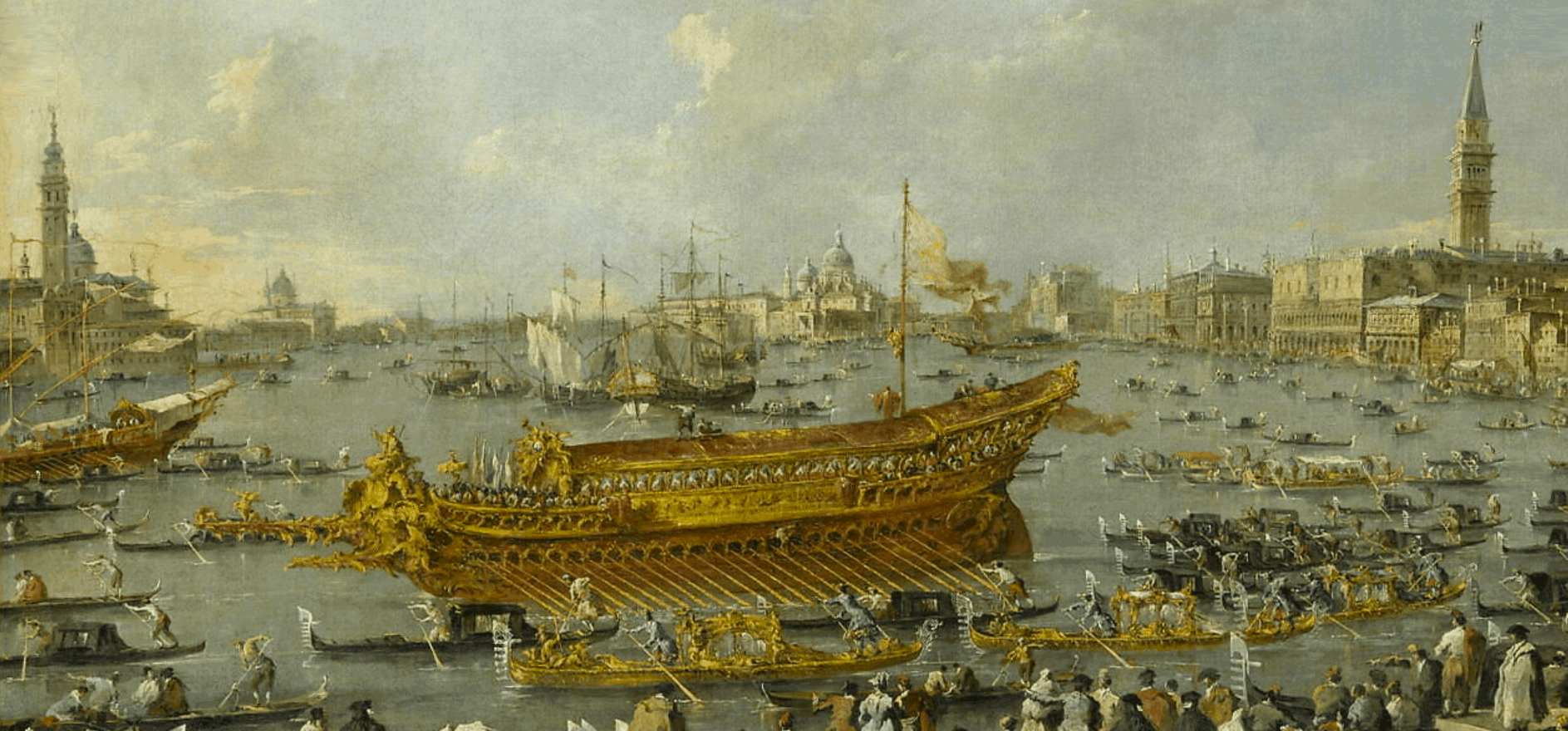The scene appears to be a realistic, oil painting of a historical maritime setting. Dominating the composition is a large, ornately decorated golden ship with a single white sail at its front. This impressive vessel is tied by numerous ropes, suggesting it is docked or otherwise anchored. Surrounding the golden boat are smaller, canoe-like boats, also seemingly crafted from gold, drawing the viewer's attention with their similar material and intricate craftsmanship.

Behind the gilded ship stand two larger sailboats, modest in comparison, with brown hulls and white sails. The water is populated with various other boats, enhancing the bustling, navigational atmosphere of the scene.

Flanking either side of the waterway are tall, stately buildings that add to the historic ambiance of the image. Notably, a large, imposing structure resides on the right side of the painting. The sky overhead is overcast, with dark clouds hinting at impending inclement weather, which adds a dramatic backdrop to this old-time maritime tableau.